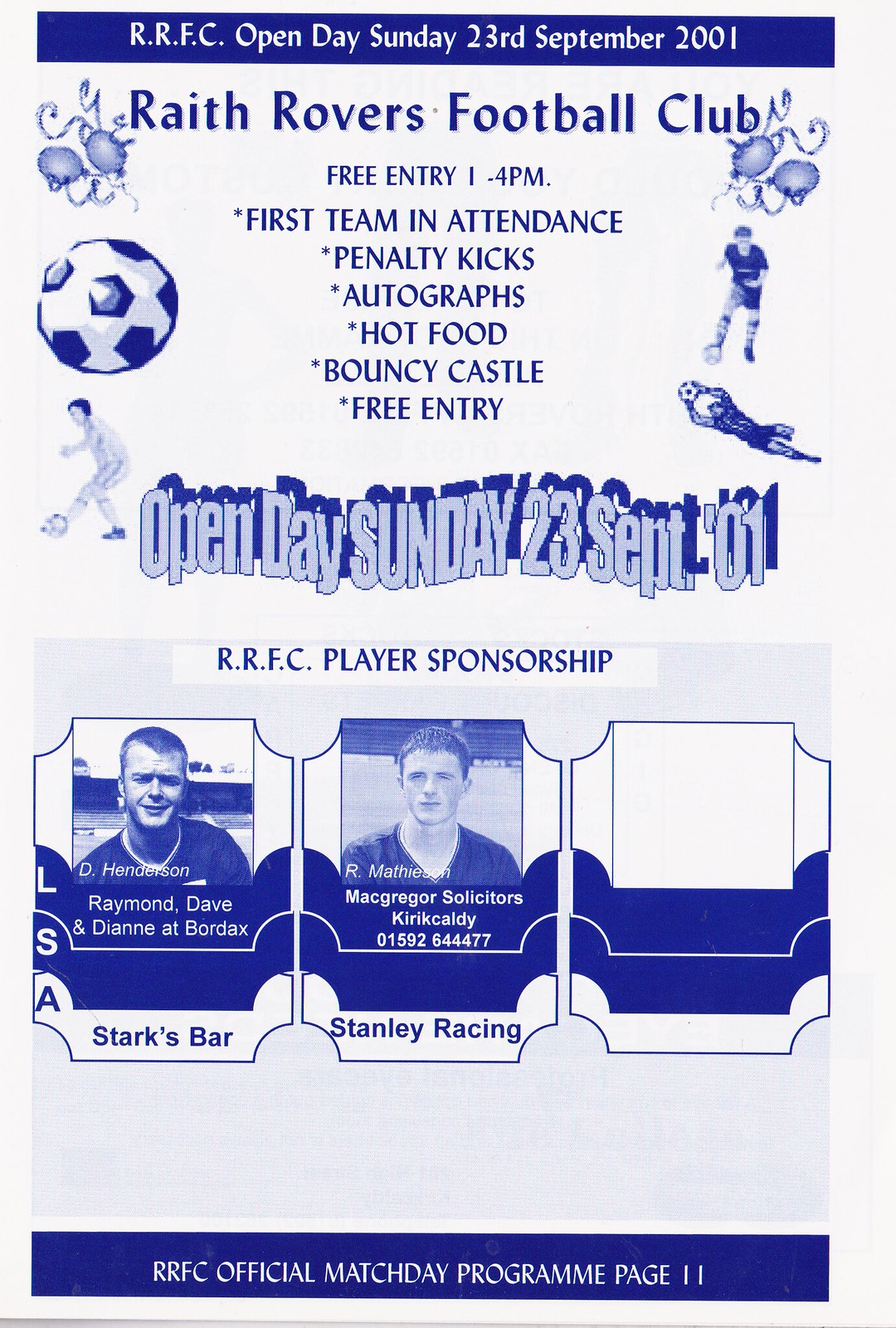The image depicts a detailed advertisement for an RRFC (Raith Rovers Football Club) Open Day event taking place on Sunday, 23rd September 2001, from 1 p.m. to 4 p.m., with free entry. The flyer has a predominant color scheme of blue text on a white background with decorative dark blue borders at the top and bottom. Promotional details include activities like penalty kicks, autographs, hot food, a bouncy castle, and the first team being in attendance. 

The visual design includes festive elements such as ribbons and balloons, alongside soccer imagery like soccer balls and players. Prominent sponsors mentioned are Stanley's Racing and Starks Bar, while the bottom of the flyer highlights a section for RRFC Player Sponsorship, displaying images of some players—though one slot appears blank. It also lists additional contributors like McGregor Solicitors and Kirkcaldy. The advertisement is part of the RRFC Official Match Day Program, specifically noted on page 11. The contact number provided is 01592 644477.